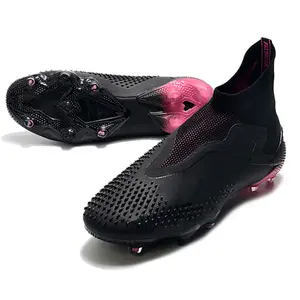This image showcases a pair of sleek black women's slip-on shoes with a rubber exterior. The shoes feature a distinctive design, including vibrant pink soles that add a pop of color to the otherwise monochromatic look. The soles are designed with small, rounded bumps that provide excellent traction, ensuring a secure grip on various surfaces. These bumps resemble tiny pink beads that stud the entire underside of the shoes, creating a textured, bumpy pattern. Perfect for casual wear, these stylish shoes combine functionality and fashion, offering both comfort and elegance in a convenient pull-on design.